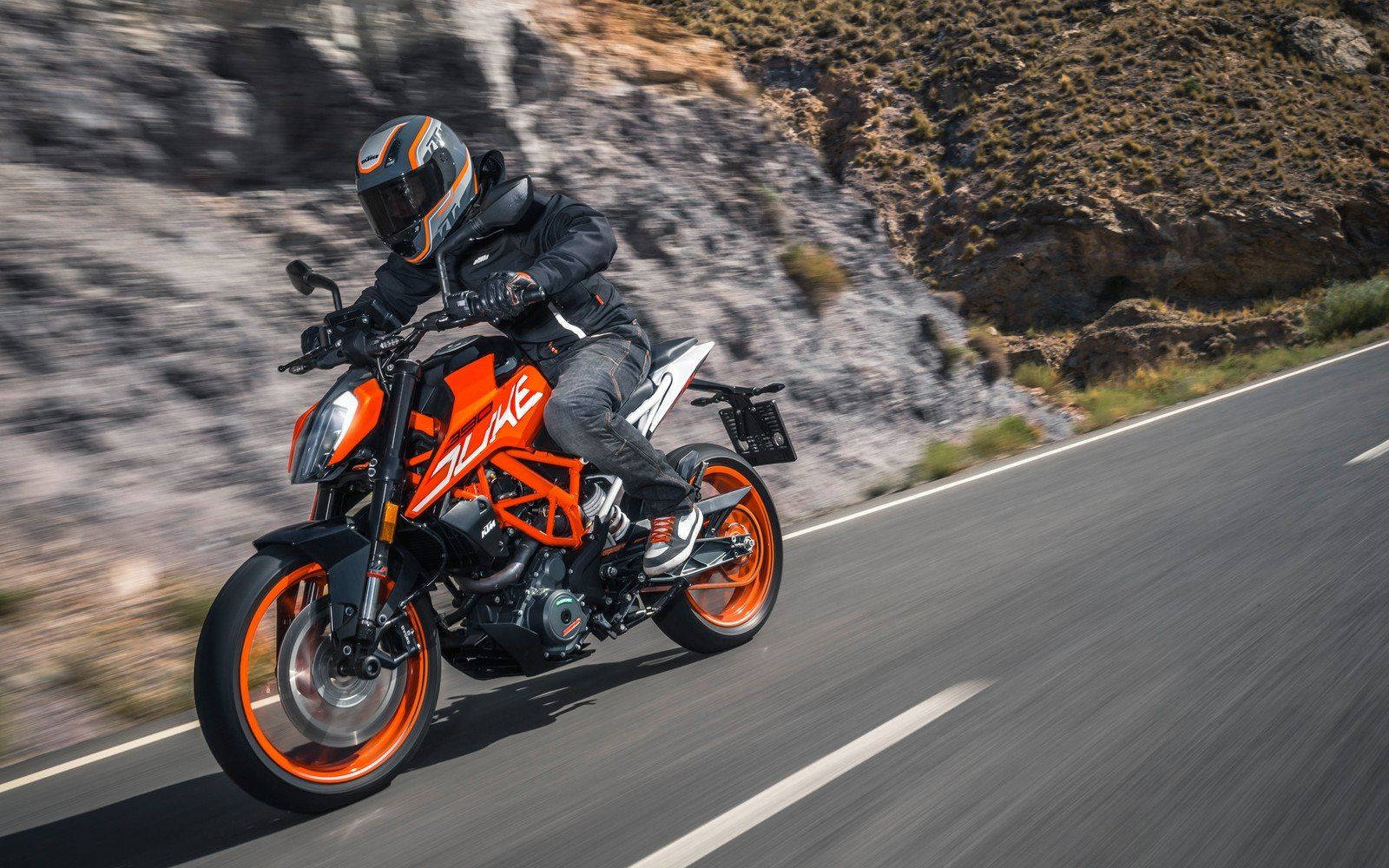A high-speed action shot captures a motorcycle rider in focus, zooming down a highway while the background blurs into a dizzying swirl of color. The rider is on an eye-catching orange and black motorcycle, with "Duke" emblazoned on its side. They are geared up in a black jacket, grayish-black pants, and sneakers with a mix of white, gray, and red laces, coordinating stylishly with their black helmet featuring orange and gray details. The pavement under the motorcycle displays streaks of movement, accentuating the sense of speed. In the backdrop, a large, blurred, gray rock formation contributes to the sense of motion, while a brown-textured rock can be seen in the upper right corner, suggesting a desert-like environment with sparse vegetation. The entire scene combines to convey the thrill and rush of high-speed adventure.